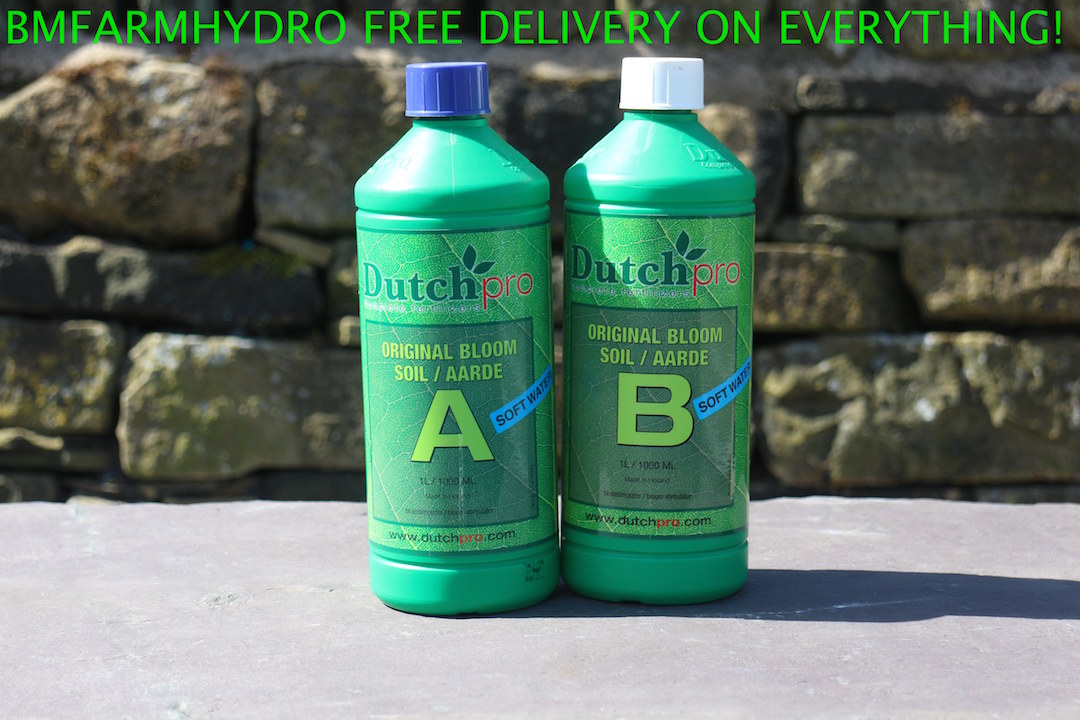The image appears to be an advertisement for horticultural products from BM Farm Hydro, prominently featuring the text "BM Farm Hydro, free delivery on everything!" in a bright green font at the top. Below the text, two green plastic bottles from the brand Dutch Pro are centered in the image. Each bottle differs slightly; the one on the left has a blue cap and is labeled "Original Bloom Soil A," while the one on the right has a white cap and is labeled "Original Bloom Soil B." Both labels also mention "soft water." The bottles are situated in an outdoor setting, with a flagstone or exposed stone wall in the background and a concrete surface below. The promotional nature and the detailed product labeling suggest these are soil enhancers or fertilizers designed for gardening or horticulture.